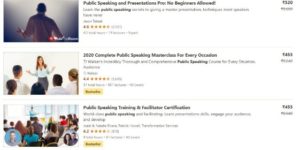The image is a composite consisting of three vertically stacked sections, each containing a photograph followed by a textual description to its right. 

In the first section, the photograph captures the upper body of a man from behind, from the waist up. His left arm is extended to his side, while his right arm's position is unclear. The accompanying text reads "Public Speaking and Presentations for Beginners," followed by a price and a descriptive paragraph with star ratings.

The second section features a woman in a white long-sleeve shirt and a gray skirt, facing forward. Five people are seated in front of her, shown from the back as they look towards her. The text next to this image includes the words "Public Speaking" along with additional details.

The third section depicts an individual standing behind a podium, addressing a classroom full of seated attendees. The text indicates that this too pertains to public speaking.